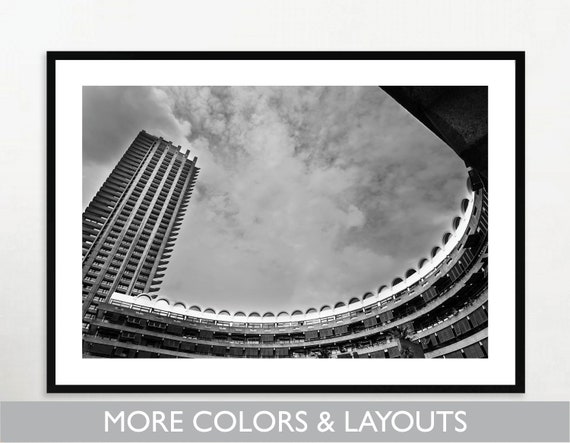In this image, a black and white photograph is displayed in a rectangular black frame with a white mat. The photograph features a strikingly tall skyscraper, captured from its base looking upward, with a clear view of clouds in the sky above. To the right of the skyscraper and spanning only three or four floors high, a curved structure, possibly part of a stadium or a separate building, is prominently visible. The image includes a footer in dark gray with white, all-caps text that reads "MORE COLORS AND LAYOUTS." The overall impression is of a thoughtfully composed architectural scene set against a dramatic, possibly cloudy sky, meticulously framed to emphasize the vertical grandeur of the skyscraper and the contrasting curve of the adjacent structure.